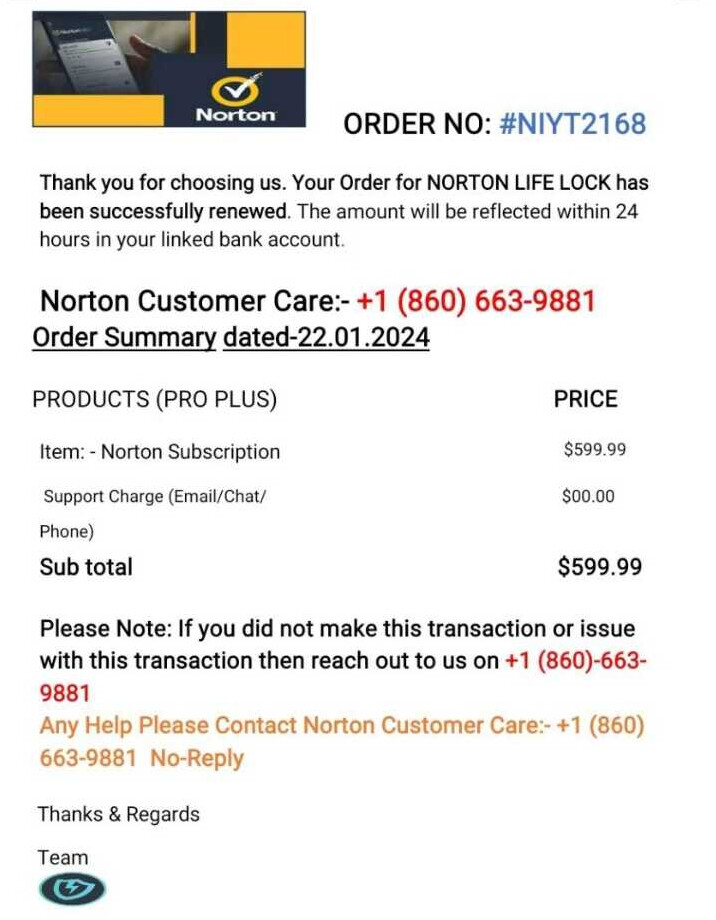In the image, the top right corner depicts a person intently looking at their phone, possibly scrolling through various pieces of information related to Norton. Below this, an organized layout of details is displayed, accompanied by several visual elements.

On the bottom right, there's an orange circle with a white checkmark inside, next to the text "Norton" in white font. To the right of this circle, the term "ORDER NO" is prominently displayed in all caps in black, followed by an actual order number in blue. Below this, a message reads, "Thanks for choosing us. Your order for Norton LifeLock has been successfully renewed. This amount will be reflected within 24 hours in your bank account."

Further down, the customer care number is highlighted in red: +1-860-663-9881. Below this, the word "PRODUCTS" is capitalized and followed by "PRO PLUS" in parentheses. Adjacent to it, the term "PRICE" is listed. Underneath, it specifies that the Norton subscription costs $599, which is noted as quite an expensive amount for what appears to be the Pro Plus version. The section goes on to mention in the left column, "SUPPORT CHARGE," which includes email, chat, and phone support for $0. 

The subtotal is emphasized in bold as $599.99. A disclaimer below advises that if you did not make this transaction or have any issues with it, you need to contact the same phone number provided earlier.

Below the disclaimer, in orange text, it states, "Any help, please contact the Norton customer care at 1-860-663-9881. You cannot reply to this." At the very bottom, the text signs off with "THANKS AND REGARDS" followed by "TEAM," adjacent to a blue shield icon featuring a lightning bolt. The entire document is set against a white background.